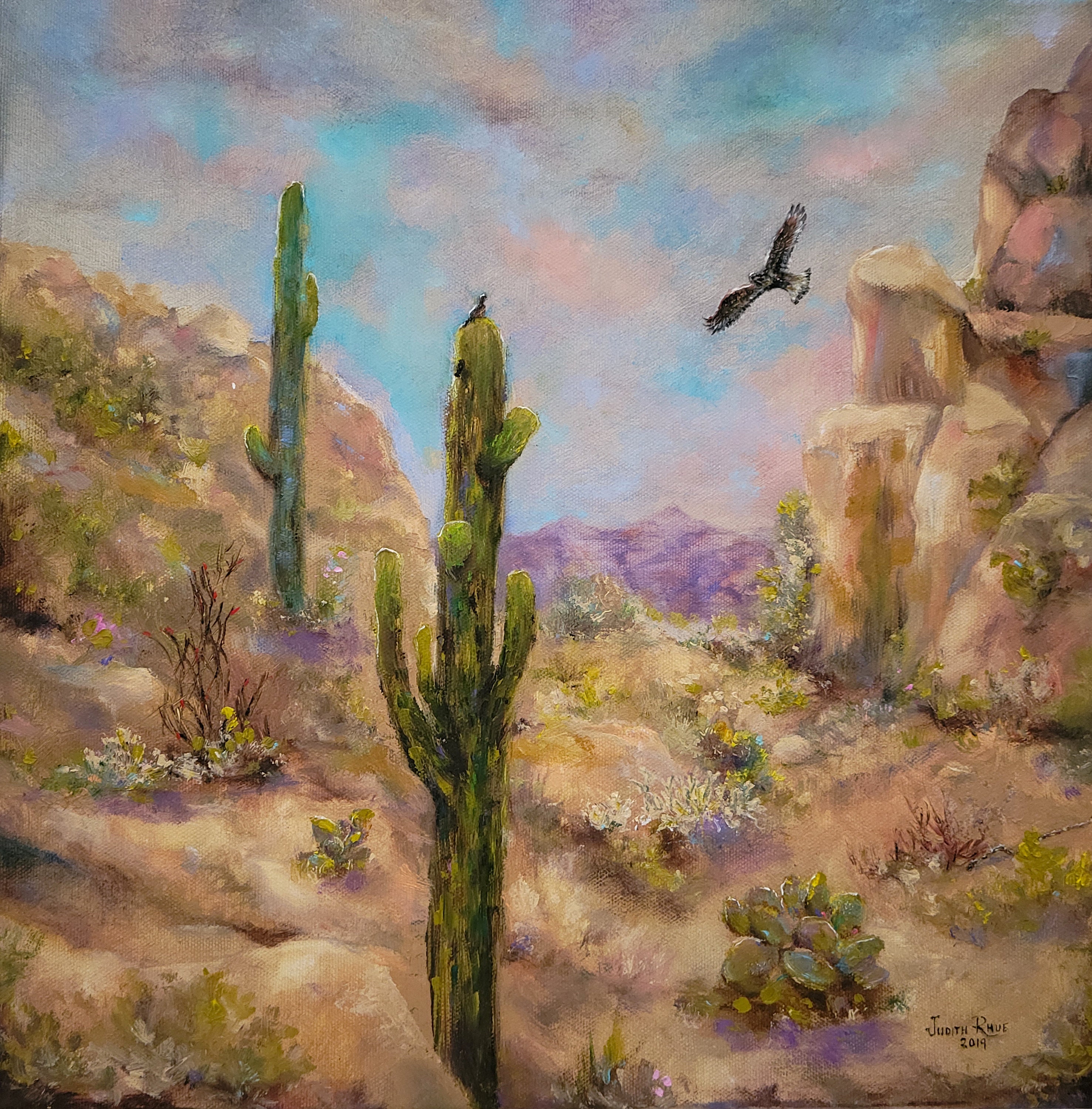This Impressionist painting depicts a detailed desert landscape characterized by a predominantly light sandy-colored or clay-like texture. The scene features two tall cactuses: one vibrant green cactus centrally placed and another slightly more turquoise-hued cactus in the background to the left. The desert ground, textured with rocky and sandy elements, slopes upward on both sides, forming gentle hills. The right slope is marked by a larger rock structure of the same tan hue as the ground. Scattered across the scene are small green plants, wildflowers, and patches of grassy thickets. In the background lies a majestic purple mountain range under a light blue sky tinged with gray clouds. Adding life to the scene, a bird with black and white plumage, possibly a falcon or vulture, flies gracefully to the left of the rocky structure, beneath the subtly clouded sky.